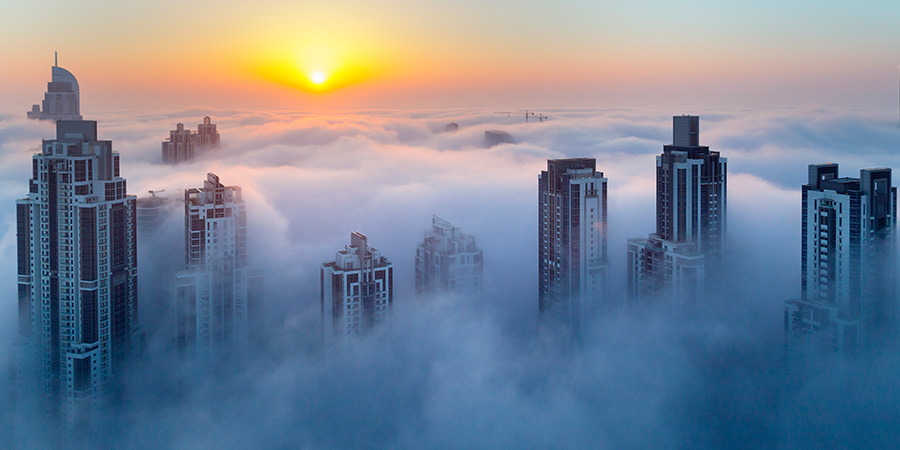This captivating image depicts a futuristic city skyline immersed in a dense blanket of fog at dusk. The sky at the top transitions from deep blue to a radiant yellow and pinkish hue near the horizon, indicative of an impending sunset. The ground is entirely obscured by dense fog, leaving only parts of the tallest buildings visible, creating an ethereal, almost otherworldly effect. 

In the foreground, seven prominent skyscrapers come into focus. On the left, a large glass-paneled building stands out, partially enveloped in the fog. Next to it is a slightly shorter building, also shrouded in mist. Further to the right are two identical buildings of equal height; the one closer to the center is more visible, while the other is almost completely obscured by the fog. Continuing rightwards, another building emerges from the fog, with a black top and silver bottom; behind it, only partially visible, is another structure. Finally, a distinct black and white building punctuates the far right of the image.

The remaining buildings in the background are barely discernible, poking through the fog like distant sentinels. The fog creates an illusion of floating skyscrapers, their tops bathed in the soft glow of the setting sun. The overall scene suggests a vantage point from one of the highest buildings, offering a breathtaking view akin to floating above the clouds. The uniform grey, black, and white palette of the buildings, coupled with the sight of the emerging sun, evokes a sense of early morning serenity and the vertical majesty often associated with major metropolitan business districts.